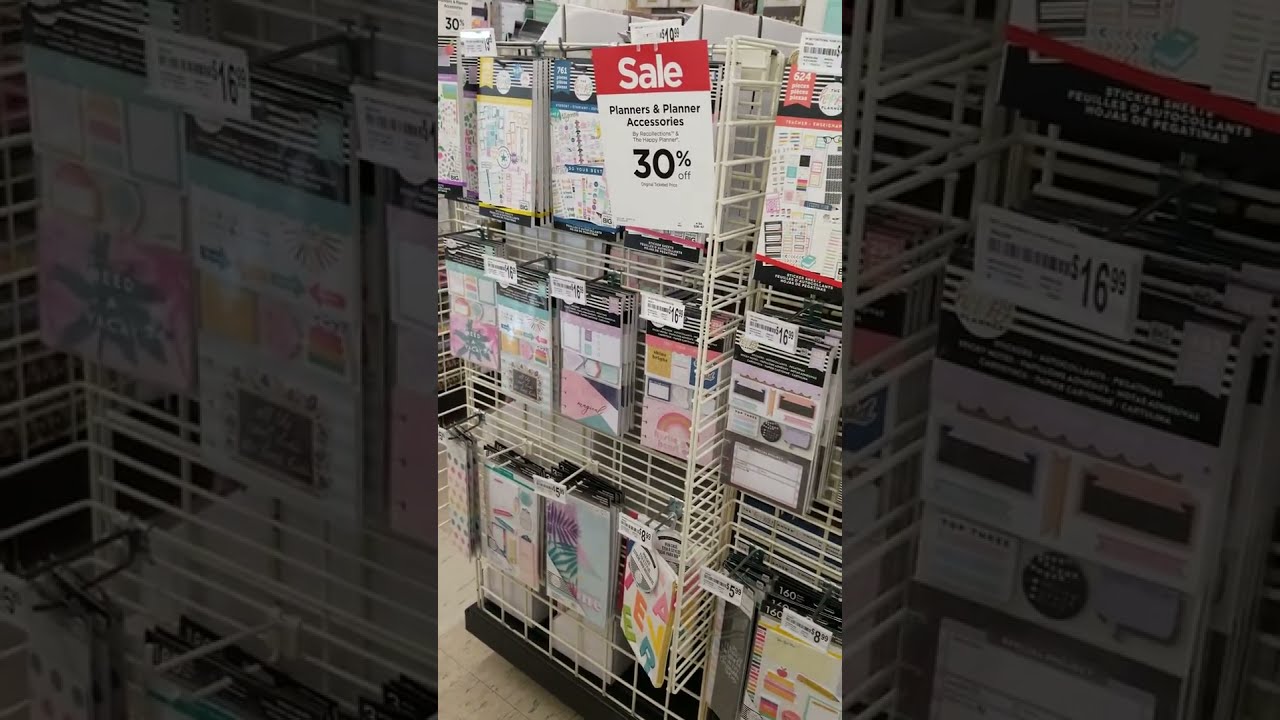The photo, taken indoors, shows movable shelving units on black caster bases, suggesting they can be repositioned throughout a store. The shelves are constructed from a flimsy white metal crate, displaying a variety of items stacked on the shelves and hanging on the sides. Prominently displayed are planners and planner accessories, with various colors visible, predominantly pink, yellow, blue, and white. These items come with individual price tags such as $5.99, $8.99, $16.99, and $19.99. A red sign with a bold "Sale" written at the top and "Planners and Planner Accessories 30% off" highlights the ongoing discount. The general impression of the setting is a retail space, possibly a craft or office supply store, featuring removable display units providing flexible product arrangement.